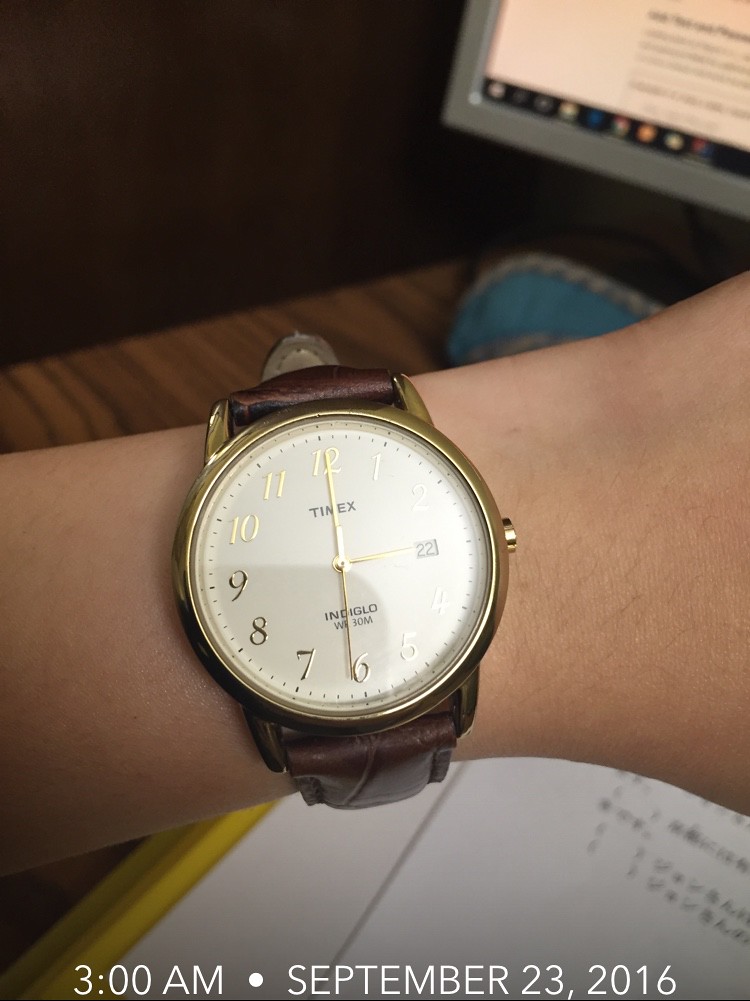In this image, a Timex wristwatch is prominently displayed on a person's left wrist, which has very light, likely Caucasian skin. The watch, indicating the time is precisely 6 o'clock, boasts a large face encased in a brass-like material with a yellowish tint and is complemented by a brown leather band. The background reveals a laminate-topped wood table adorned with a textbook and some yellow folders. The top right corner of the image captures the base of a computer screen, beneath which is a mysterious black and turquoise object. An inscription at the bottom of the image reads "3 a.m. September 23, 2016."